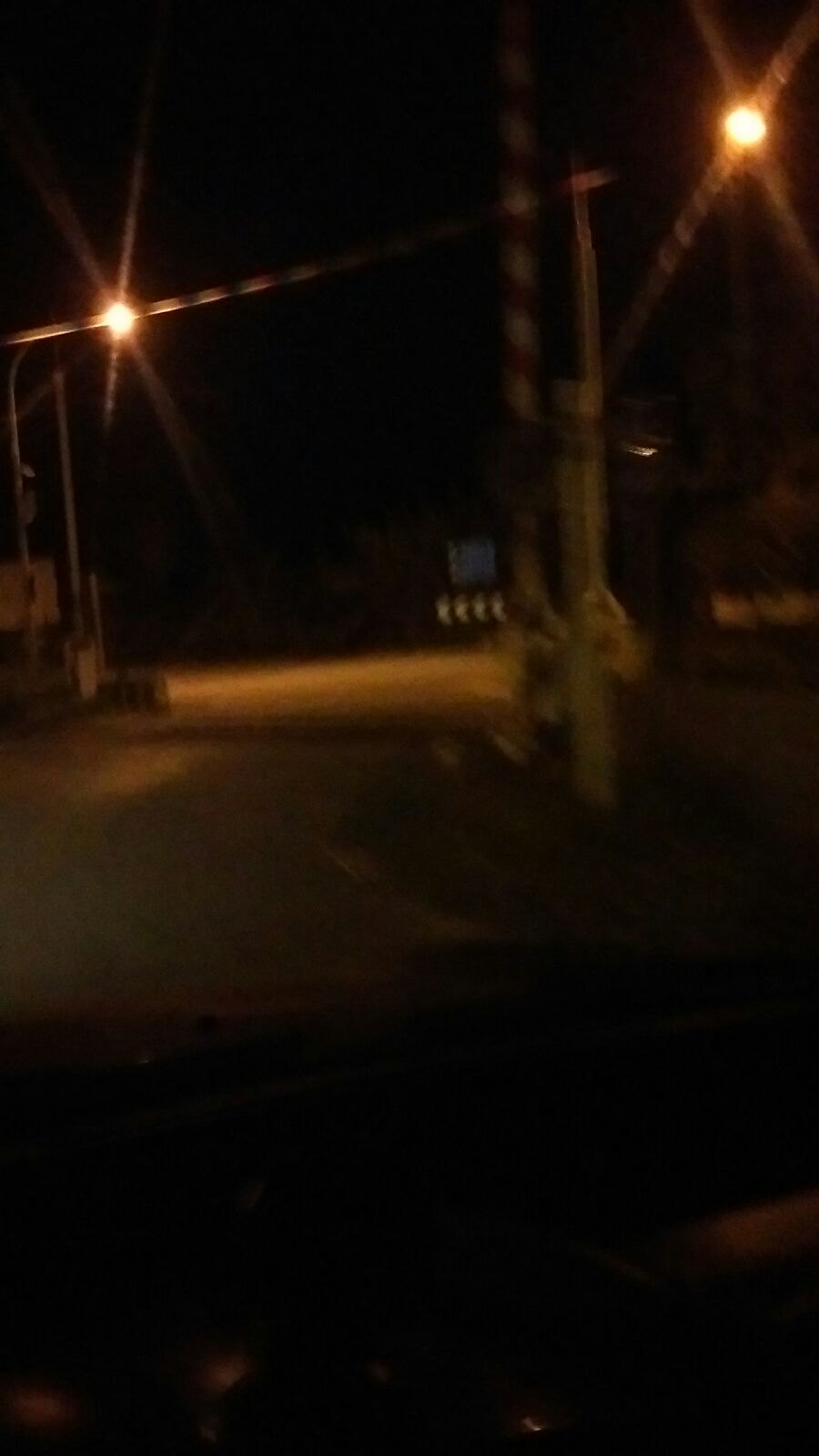An atmospheric nighttime scene likely depicting an industrial or construction site. The image captures a stark contrast between light and dark elements. In the top right corner, a glaring light illuminates part of the scene, mirrored by another glaring light on the left side. A wire is also visible on the left, perhaps signifying a suspended overhead fixture or utility line. The floor at the bottom of the image is shrouded in deep shadow, with hints of slightly illuminated brownish tones that suggest it might be made of stone or concrete.

The background is enveloped in darkness, though some indistinct objects are visible on both the left and right sides. The left side features what appear to be poles, scattered perhaps as part of the site infrastructure. Black and yellow caution markings are faintly visible in the background, indicating a safety zone or restricted area. The middle of the image remains vague and undefined, adding to the enigmatic atmosphere of the scene.